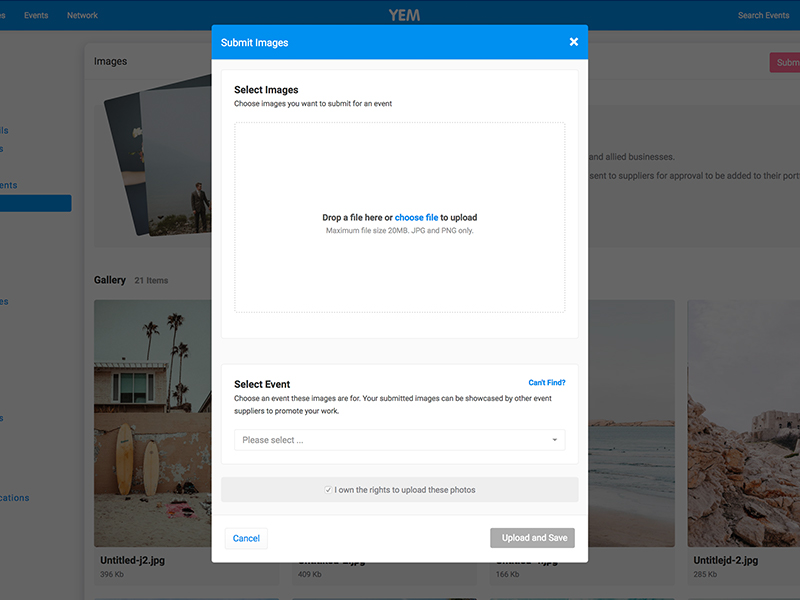This detailed screen capture showcases a complex interface with both background and overlay elements. The background image features a grayed-out site and contains a blue navigation bar at the top displaying the word "Events" in white text, partially obscured by adjacent menu options such as "Network" and "YEM" in all caps. On the other end of this bar, it reads "Search Events".

Beneath the navigation bar, a black text heading "Images" appears, followed by two photographs. The first photo is indistinct, showing only black and white colors. The second photo features a man in a suit, though details are not clear. Adjacent to these images, partially visible black text likely reads, “Allied Businesses: Sent to Suppliers for Approval,” but the rest of the text is cut off. Additionally, a partial view of a submenu nearby includes some blue text and a blue box, but most of it is nearly cut off.

Further down, the text "Gallery, 21 Items" is displayed, along with a beach scene featuring an array of surfboards leaning against a rough, tan retaining wall with visible damage. Accompanying this scene are white sand, scattered shoes, and towels. Palm trees and a tan house with a white window frame are visible in the background. Additional images include a beach with waves and a photograph labeled “Untitled.jpeg,” depicting an assortment of rocks.

An overlay screen pop-up overlays this background, dominated by a blue bar with white text reading "Submit Images" and an 'X' for closing the pop-up. Below this is the text "Select Images" in black, instructing users to choose images for submission for an event. A large white box follows, containing drop-zone instructions in black and blue text: "Drop a file here or choose file to upload," specifying a maximum file size of 20 MB for JPEG and PNG formats.

Further directives in black text read "Select Event," advising users to choose an applicable event for their images, noting that submitted images can be showcased by other event suppliers to promote the user's work. Beside this is a blue text link reading "Can't Find" and a pull-down menu marked "Please Select." At the bottom, gray text reads, "I own the rights to upload these photos" with an associated checkbox. The pop-up concludes with two buttons: a blue "Cancel" button and a gray and white "Upload and Save" button.